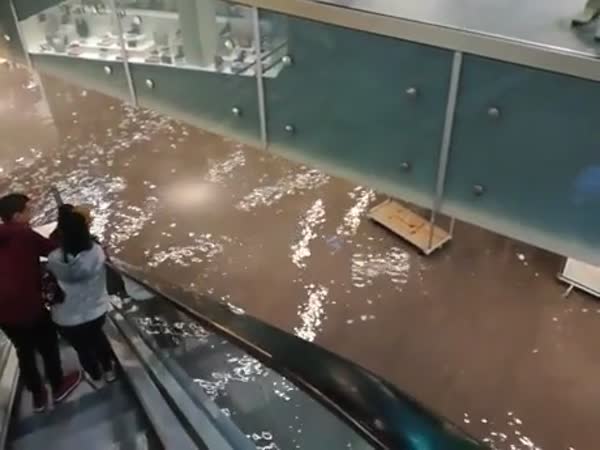The photograph captures a scene inside a shopping mall from the top of an escalator angled downward. In the lower left part of the image, two people are descending the escalator. On the right, a man dressed in a maroon hoodie, black pants, and maroon shoes stands next to a woman in a light gray hoodie, tight denim pants, and white shoes. Both individuals have black hair. A third person is visible ahead of them, but details are indistinct.

In the upper right, the facade of a store is partially visible, showcasing a white, well-lit area that appears to contain jewelry or similar items. The floor of the mall, which appears to be flooded, is composed of a brown, reflective tile that gives the illusion of standing water. The light's reflection on the floor adds to the image's dynamic. Overall, the photograph, characterized by earthy tones and the stark contrast between the illuminated store and the seemingly flooded floor, evokes the bustling yet surreal atmosphere of a shopping mall.